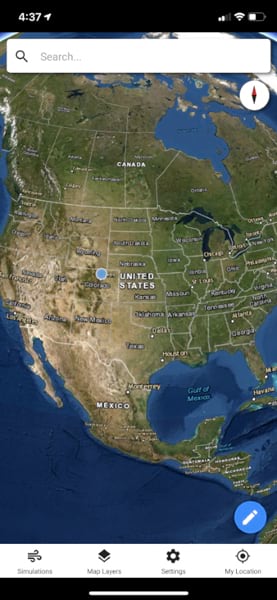The image is a vertical screenshot from a smartphone. At the top, there's a black status bar displaying the time "4:37" in white on the upper left, followed by a navigation arrow pointing northeast. On the right side of this black bar, Wi-Fi and battery icons are visible. Below the status bar, there's a white search bar with a magnifying glass icon on its left side.

The main portion of the screen is occupied by a detailed map. The map covers parts of North America including the United States, Canada, Mexico, and Central America, showcasing green and brown land areas against blue waters. The countries are clearly labeled, with Canada, the United States, and Mexico among them.

Beneath the search bar, slightly towards the right, there's a white circular icon featuring a directional symbol pointing north. In the bottom right corner of the map, there is a blue circular button with a white pencil icon inside it. At the very bottom of the screen, there's a white navigation bar that includes several options: "Simulations," "Map Layers," "Settings," and "My Location," each represented by corresponding symbols.